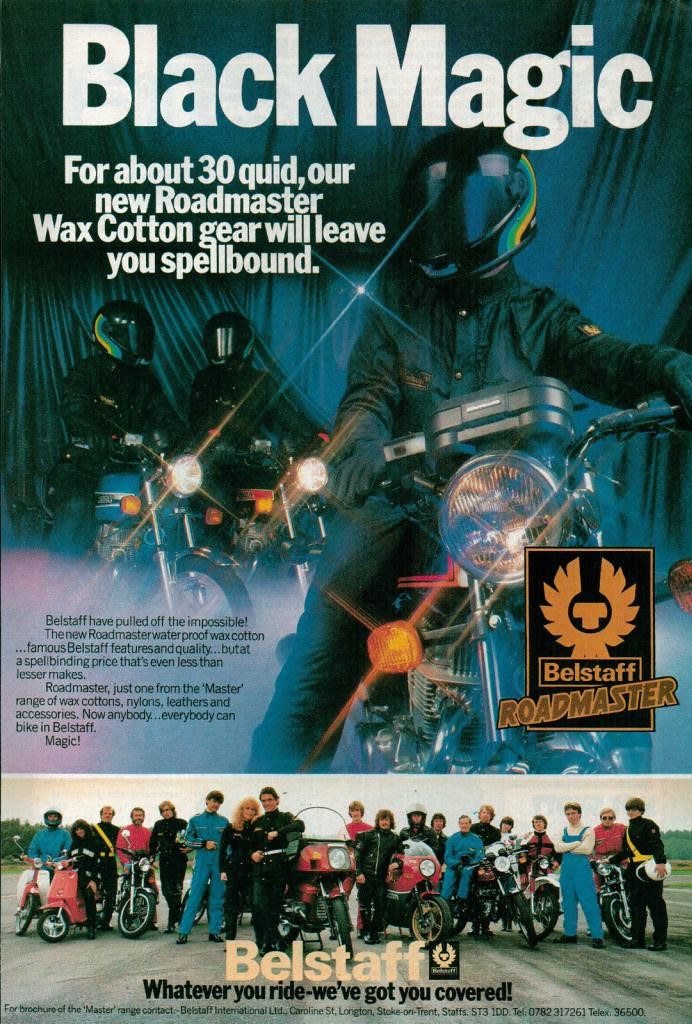This is a professionally crafted advertisement showcasing the new Bell Staff Roadmaster wax cotton gear, highlighted with a sophisticated and stylish layout predominantly featuring shades of black, blue, yellow, red, and hints of purple. The top of the ad captures the tagline in white font: "Black magic for about 30 quid. Our new Roadmaster wax cotton gear will leave you spellbound." Beneath this, a striking image displays three helmeted motorcyclists dressed in uniform motorcycle apparel, with the rider in the front standing out prominently in dark green. Behind him, two other riders on motorcycles form a dynamic backdrop.

The bottom section of the advert reveals a gathering of approximately 15 bikers of varying heights and ages, all standing by their motorcycles and facing the camera, emphasizing the gear's broad appeal. Splashed across this image are the words: "Bell Staff. Whatever you ride, we've got you covered." To the right, in the lower-middle portion, additional text accentuates Bell Staff's commitment to delivering unmatched quality: "Bell staff have pulled off the impossible. The new Roadmaster waterproof wax cotton boasts famous Bell staff features and quality at a spellbinding price even less than lesser makes." Accompanying this text is the notable Bell Staff Roadmaster logo in bold orange and black, reaffirming the brand's prestige and legacy in the motorcycling community.